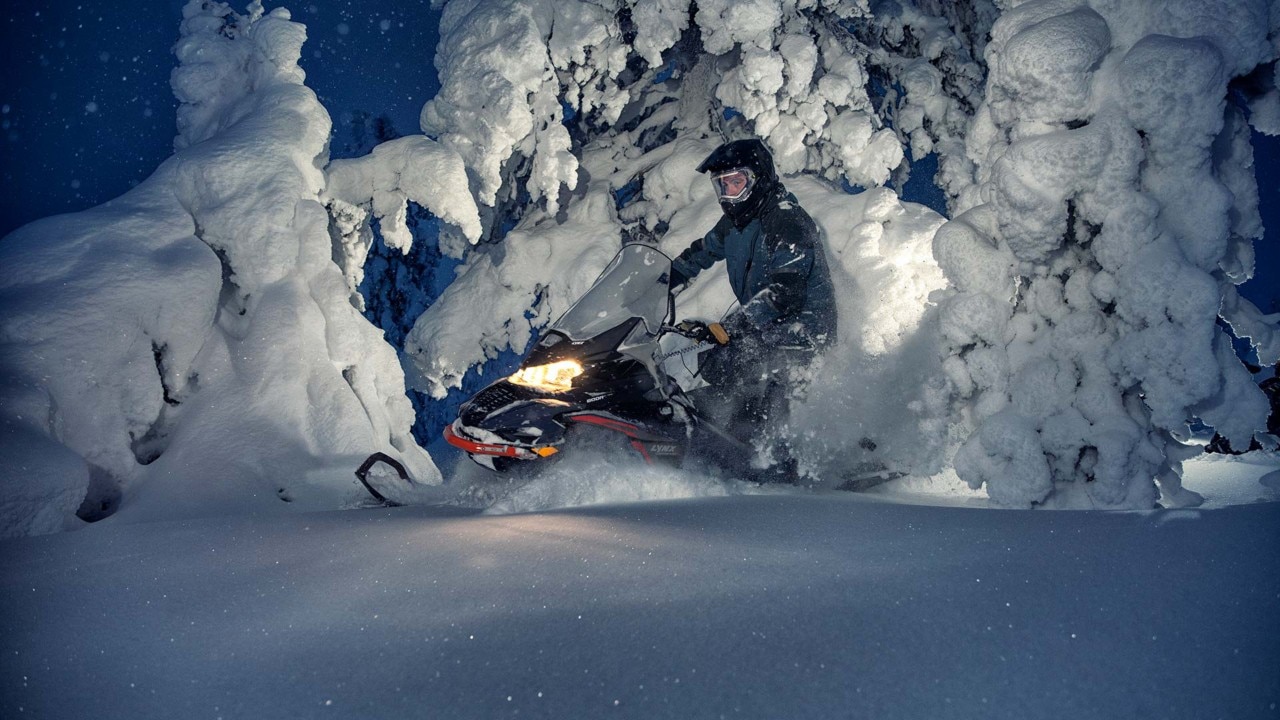A color photograph, in landscape orientation, captures a dynamic nighttime winter scene. The focus is on a person driving a black and red snowmobile across a snow-covered landscape. They are clad in a blue and black jacket, with a black helmet featuring a visor, and amid a swirling flurry of snow kicked up by the snowmobile. The headlight on the machine is illuminated, contrasting against the darkening blue sky above, speckled with a few stars. The entire landscape is blanketed in thick snow, heavily coating the ground and trees, which extend from the foreground into the background. Snow continues to fall, adding to the serene but chilly atmosphere of the scene likely set in a northern region such as Alaska. The photograph exudes an essence of representational realism, perfectly capturing the silent beauty and activity of this wintery outdoor setting.